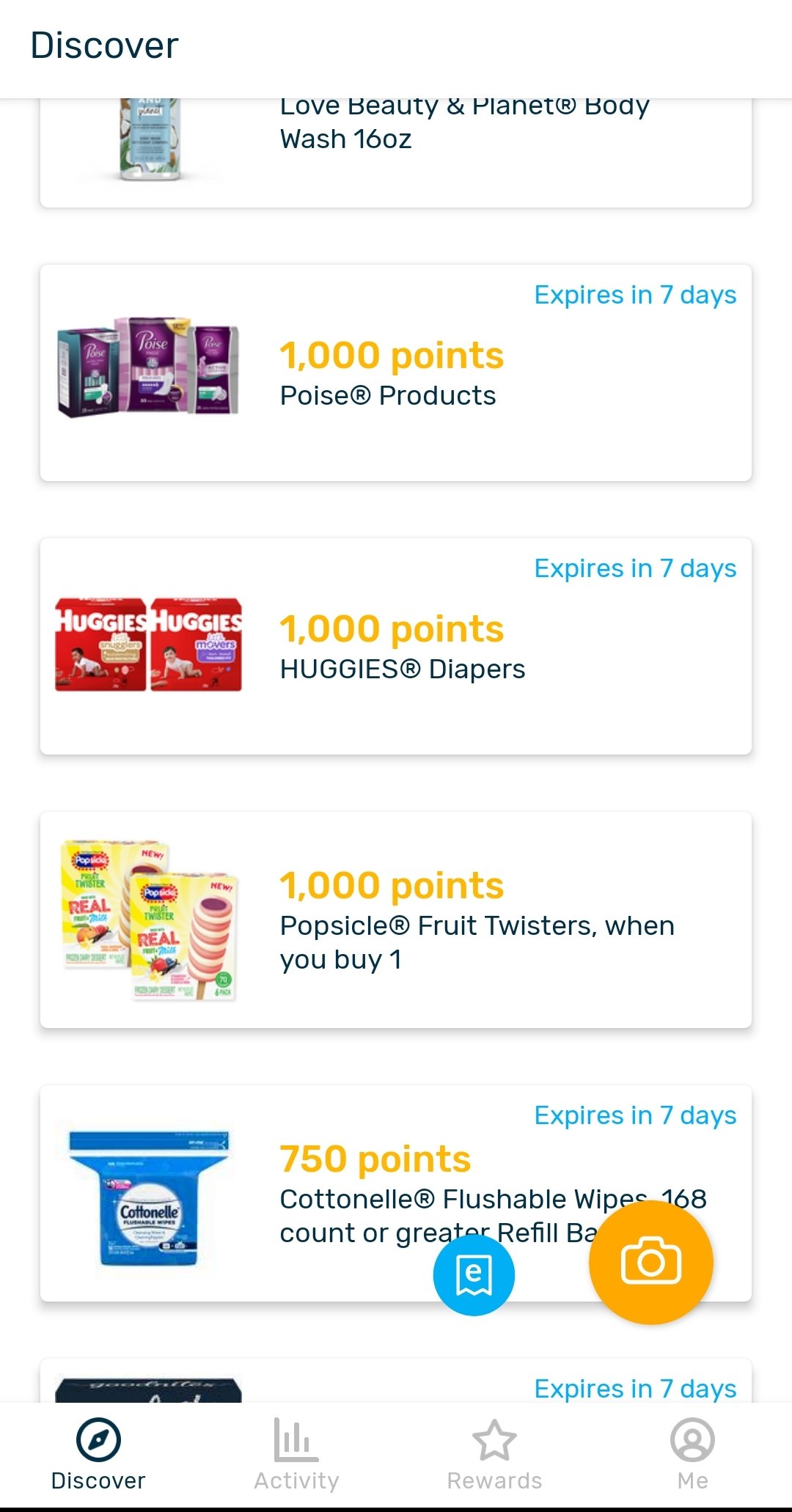The image appears to be a screenshot of a smartphone displaying a rewards app interface. The app allows users to earn points for purchasing various products, which can then be redeemed for gift cards or cash. The screen has a white background with several rows featuring different products, each enclosed in white boxes.

At the top of the screen, the word "Discover" is prominently displayed in dark blue text. Below this header, the app lists products in rows. The first product is a "Love Beauty and Planet Body Wash, 16 ounces," accompanied by an image of the body wash. Next, there’s a row for "Poise Products," showcasing an image and offering 1,000 points, with a note that this offer expires in seven days.

Following this, there is a photo of two Huggies diaper packages, also offering 1,000 points and expiring in seven days. Below this, the app features "Popsicle Fruit Twisters," which earn the user 1,000 points when one is bought. Finally, the last listed product is "Cottonelle Flushable Wipes, 168 count or greater refill," worth 750 points.

At the bottom of the screen, there are two icons; a yellow camera icon for taking photos and a blue icon for submitting e-receipts. The navigation bar at the bottom of the screen includes options labeled "Discover," "Activity," "Rewards," and "Me." The "Discover" option is highlighted in dark blue, indicating the current screen, while the other options are in light gray.

Overall, this app provides a scrolling list of products through which users can discover various rewards.